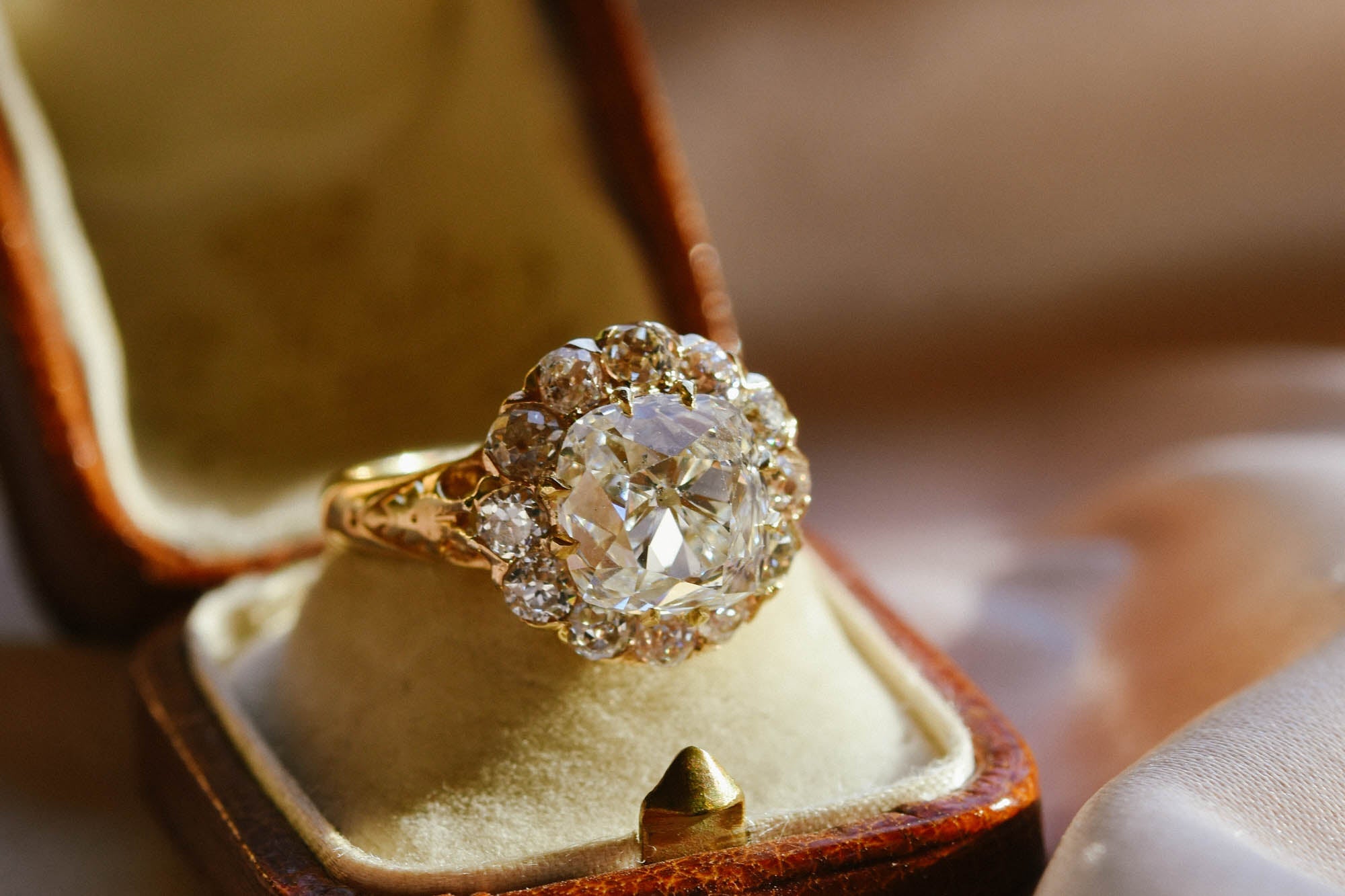This image captures a detailed view of a luxurious gold ring prominently placed inside an antique-looking jewellery ring box. The ring, situated at the center of the composition, boasts a large central diamond encircled by twelve smaller diamonds, all securely held by intricate gold detailing. The ring itself has a gold band that glistens under the light. The case that houses this exquisite piece is made of chestnut brown leather, exhibiting a slightly worn, vintage appearance, suggesting its age. The interior of the box features a cream-colored, velvety lining, which provides a soft, elegant backdrop for the ring. The box, approximately 2x2 inches in size, is open with its lid flipped back, drawing attention to the ring within. The background of the photograph is blurred, keeping the focus entirely on the ring and the detailing of the box.